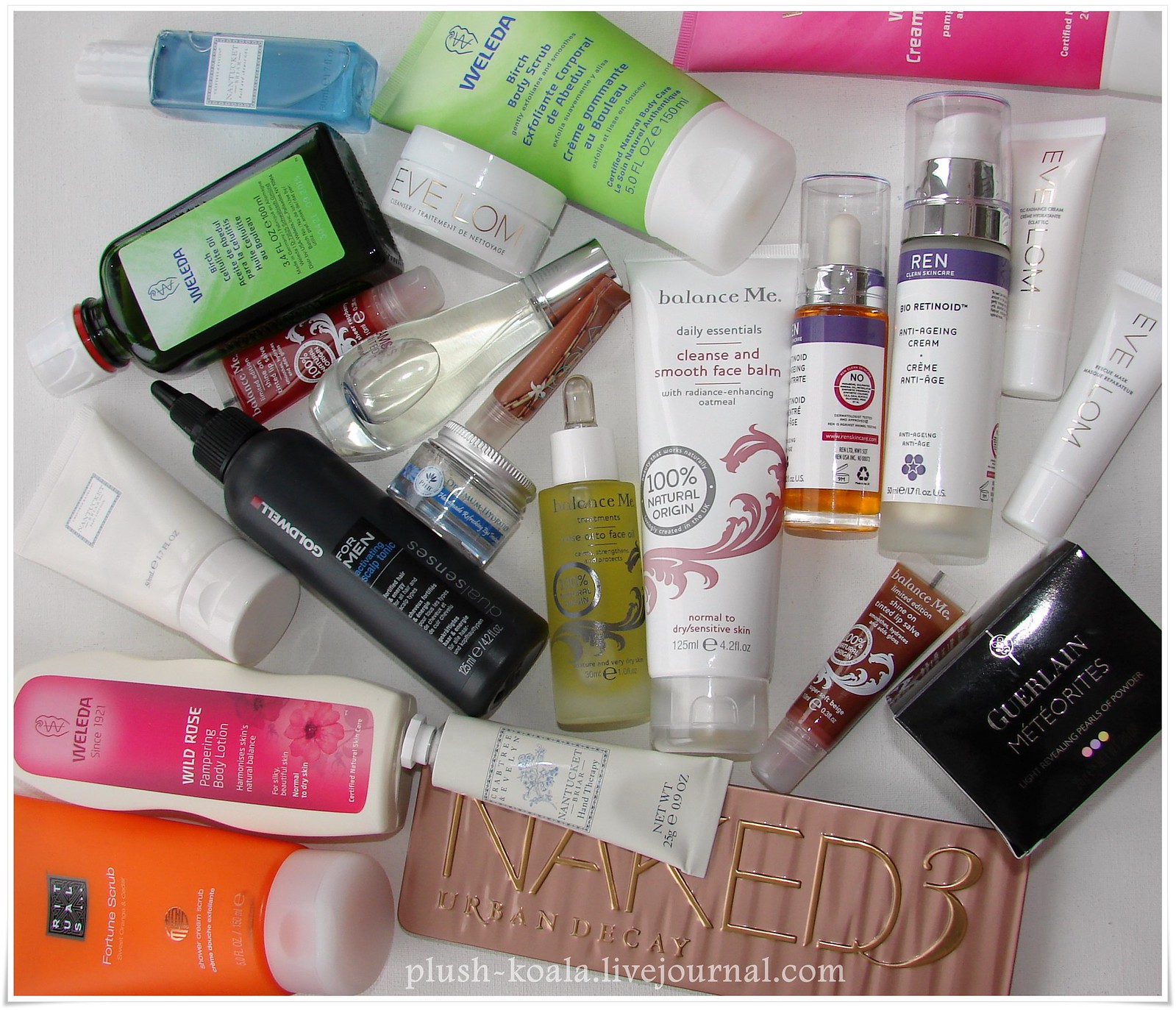The image captures a cluttered assortment of around 10 to 15 skincare products arranged haphazardly on a white countertop. Overlaid at the bottom of the picture is white text reading "plush-koala.livejournal.com," indicating that the image originates from a LiveJournal account. 

The diverse collection includes items ranging from small chapstick tubes to larger bottles of lotion and shampoo. Most of the containers are white with printed text, though some stand out in colors like orange and black. Notable brands among the array include Bio-Retinoid Anti-Aging Cream and Cleanse and Smooth Face Balm, hinting at a focus on skincare and anti-aging routines. Among the collection is a Naked Urban Decay makeup palette and a Wild Rose Pampering Body Lotion, suggesting a blend of skincare and beauty products.

Additionally, there are several organic products by brands such as Weleda. The assortment features both men’s and women’s products, although the majority are aimed at women. A Rituals bottle labeled "Fortunate Scrub" is part of the men’s selection, though it is suggested that many items could be used by any gender.

While predominately skin and body care items, the collection includes minimal makeup products, focusing instead on various lotions, balms, and scrubs. The overall impression is of a meticulous and diverse skincare routine, keenly curated and varied in its offerings.